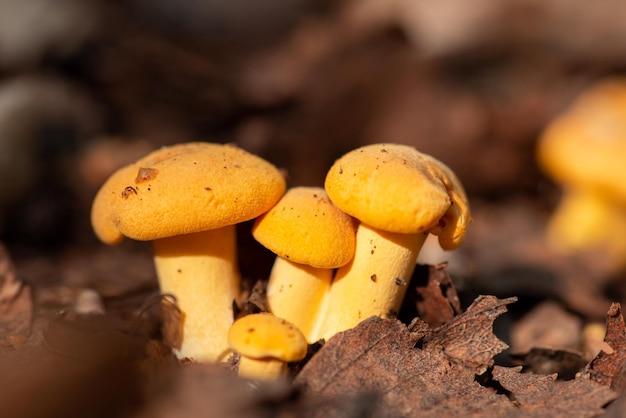This professional photograph captures a vibrant forest scene focused on a cluster of bright yellow mushrooms emerging from a bed of decomposing brown leaves. The composition features four mushrooms with large caps and moderately thick stems. On the left side, a very large mushroom stands prominently, with a slightly smaller one on the right that has a distinctive, chipped cap resembling a pac-man shape. Between these two is a shorter mushroom, and nestled in front of this trio is a miniature mushroom about a quarter of their size. The mushrooms display subtle variations in color, with the caps being a vivid golden-yellow and the bases a pale yellow, accentuated by brown speckles. The background is a soft blur of earthy browns, grays, and hints of other colors, possibly from fallen leaves or rocks, enhancing the focus on the mushrooms. To the right in the blurred background, another mushroom is faintly visible, contributing to the depth and natural setting of the image.